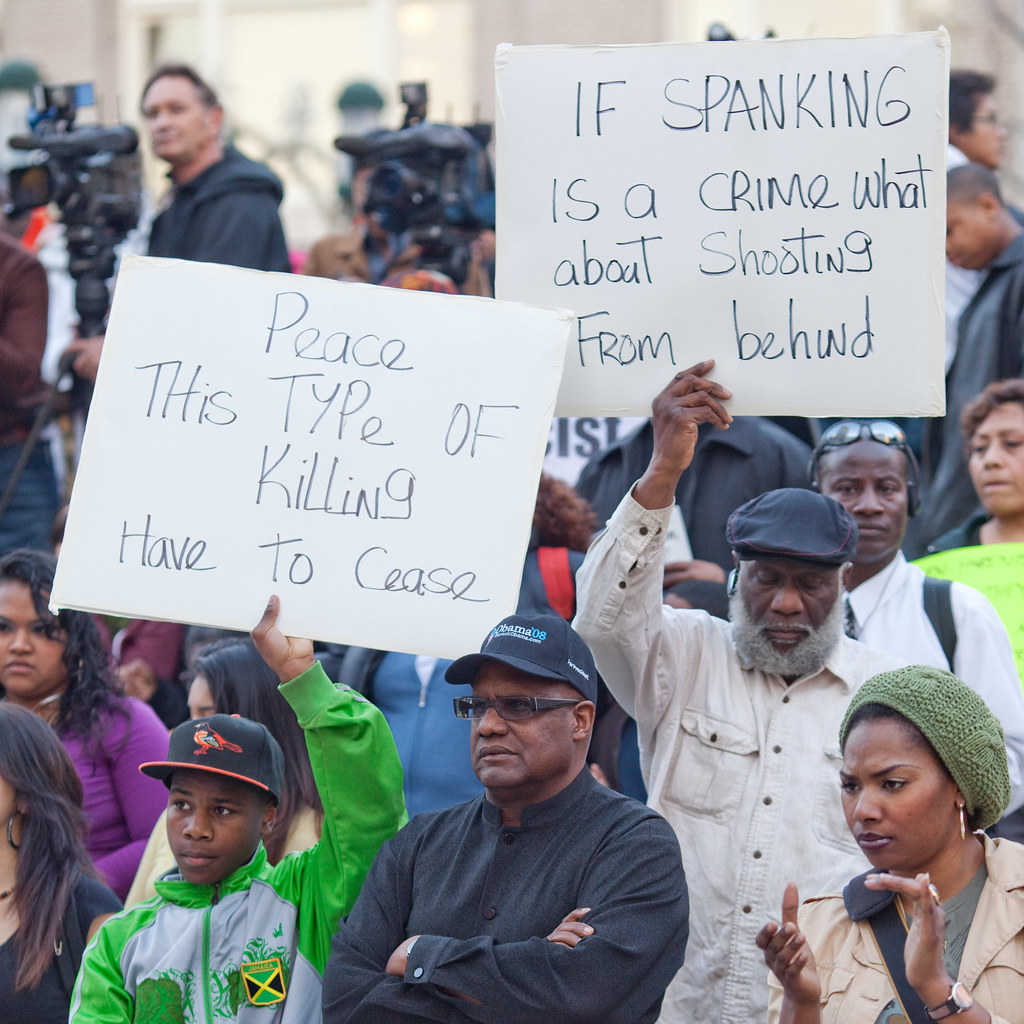The image encapsulates a poignant outdoor protest predominantly attended by African American individuals. The scene is somber, with attendees displaying expressions of stern focus as they direct their gaze towards an unseen event or figure off-camera. In the lower left-hand corner, a child dressed in a black ball cap, green and gray sweatshirt, and a shirt adorned with a bird print and a Jamaican emblem, holds a sign reading, "Peace. This type of killing has to cease." Just behind him to the right, an older man with a gray beard and a white shirt prominently displays a sign that says, "If spanking is a crime, what about shooting from behind?" The crowd, diverse yet unified in purpose, appears captivated and tense, underscoring the grave nature of the protest against violence, presumably police shootings. Despite the blurred background, news cameras are discernible, hinting at the media presence capturing this critical moment.